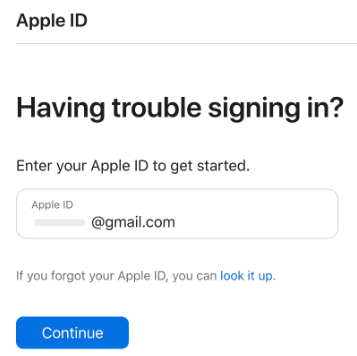A screenshot of the "Having trouble signing in?" page for Apple ID is displayed. At the top, bold black text reads: "Having trouble signing in?". Below, regular black text prompts users to enter their Apple ID to get started. The Apple ID entry field shows an email address in the format "******@gmail.com," with the first part of the email obscured by a gray box for privacy. Beneath this, there's a message stating "If you forgot your Apple ID, you can look it up," followed by a blue hyperlink labeled "look it up." At the bottom of the page, there is a blue "Continue" button. The entire interface is set against a plain white background.